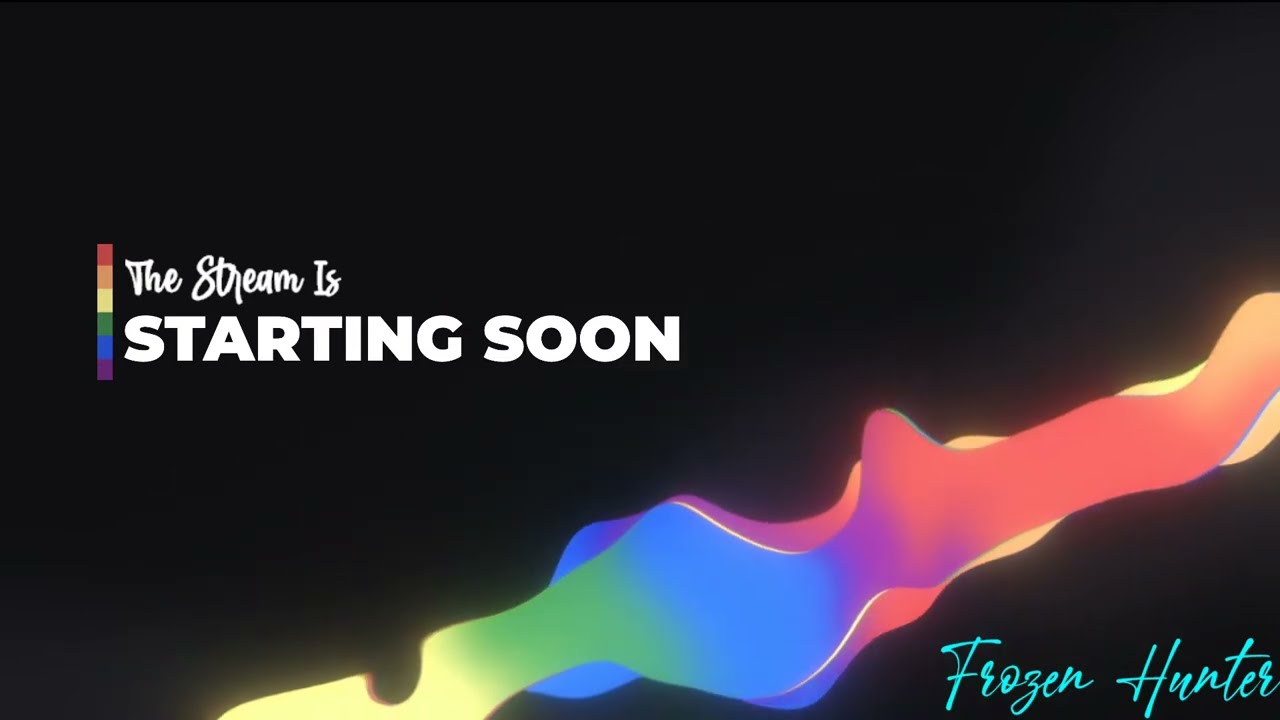The image is a promotional splash screen with a black background that features a vibrant, multicolored paint splash or nebula-like design extending diagonally from the mid-left center to the middle right edge. The colors in the splash transition from yellow to green to blue to purple to red, creating a tie-dye effect. In the vertical center of the image, there is a narrow, rainbow-colored bar with colors red, orange, yellow, green, blue, and purple. To the right of this bar, white text reads "The stream is," and underneath it, in bold sans serif font, "starting soon." In the bottom right corner, the name "Frozen Hunter" is written in a light blue cursive font.